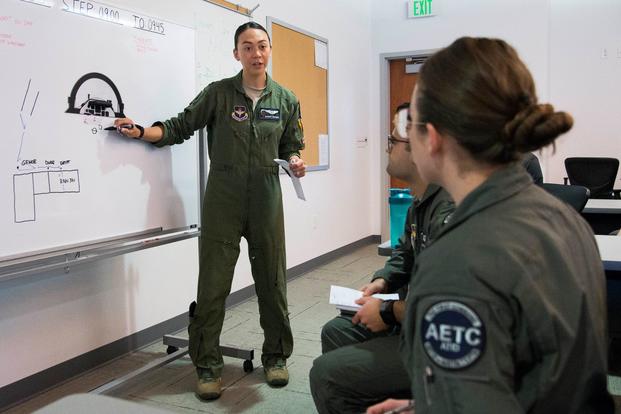In this detailed photograph taken in a classroom setting, a female instructor dressed in a military green jumpsuit is standing in front of a large whiteboard, actively engaging in a lecture by drawing images on it. In her right hand, she holds a black marker, while her left hand grips a piece of paper. Notably, she wears a black watch on her right wrist and a ring on her wedding finger. The whiteboard includes drawings that seem to resemble instruments, possibly related to military aircraft or vehicles.

In the foreground, two students can be seen. The first is a woman with brown hair tied in a bun, and she is wearing a similar green jumpsuit featuring a patch labeled "AETC." The second student is a man wearing eyeglasses, also dressed in the same military attire, suggesting a formal training session. Both students appear to be paying close attention to the instructor.

The classroom backdrop includes an exit sign above a door and a large corkboard next to it on a white wall. This and other small details like the students' brown shoes and the instructor's presentation highlight the structured, military training environment of the scene.